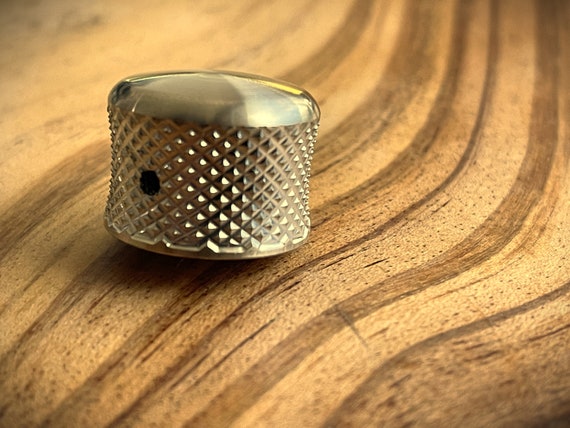In this photograph, a small, metallic object, resembling a lid, knob, or switch, is prominently featured. The object is gold in color, though not overly saturated, and positioned on a wooden surface with wavy, swirling grain patterns in light to medium brown hues. The metallic item is squat and cylindrical, with smooth, rounded top and bottom surfaces. The sides boast a textured diamond pattern, contributing to its ornate appearance. A small black or dark hole is visible on the side of the object, revealing the interior. The detailed craftsmanship of the metal piece contrasts with the natural, flowing patterns of the wooden base, making this item the focal point of the image.